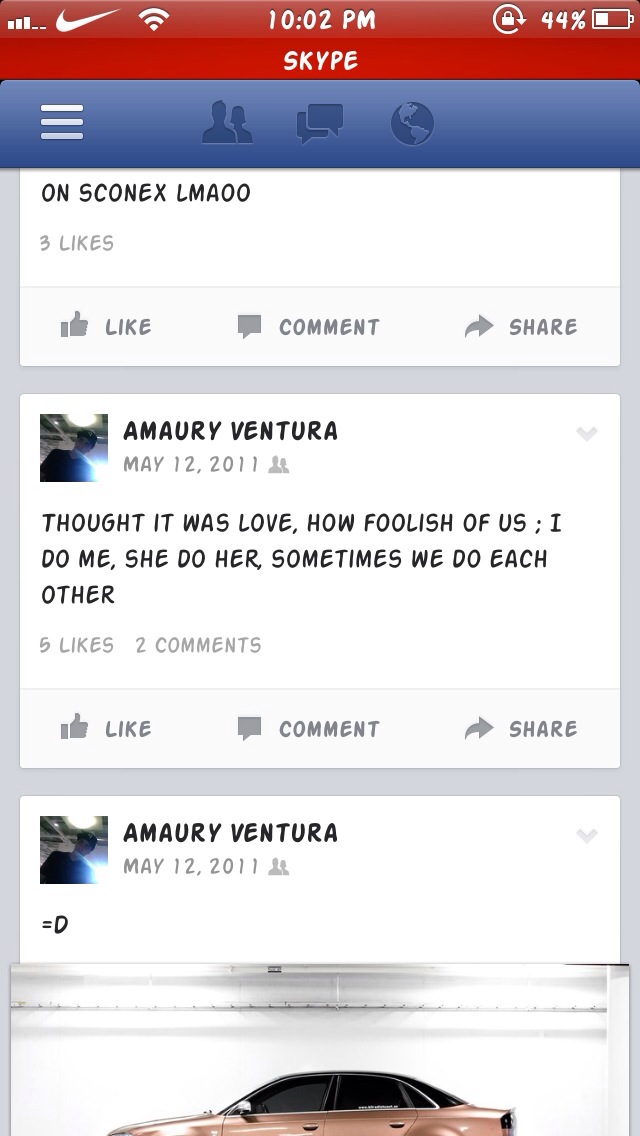The image is a detailed screenshot from a cell phone depicting a Skype interface. At the top of the screen, there is a red status bar showing cell signal strength, a Nike swoosh indicating Wi-Fi connectivity, the time reading 10:02 PM, a lock icon, and the battery level at 44%. The Skype app, which features a characteristic Comic Sans-like font, displays several posts from a user named Amari Ventura. 

The first post, dated May 12, 2011, reads: "On Skonex LMAOO" with three likes. Following this, another post by Amari Ventura from the same date states: "Thought it was love. How foolish of us. I do me. She does her. Sometimes we do each other," with five likes and two comments. A third entry from Amari Ventura features a smiley face with a tongue sticking out alongside an image of a car, described as a rose champagne-colored sedan with a black top. The interface includes various icons for people, chat, and world navigation within a white-on-blue menu.